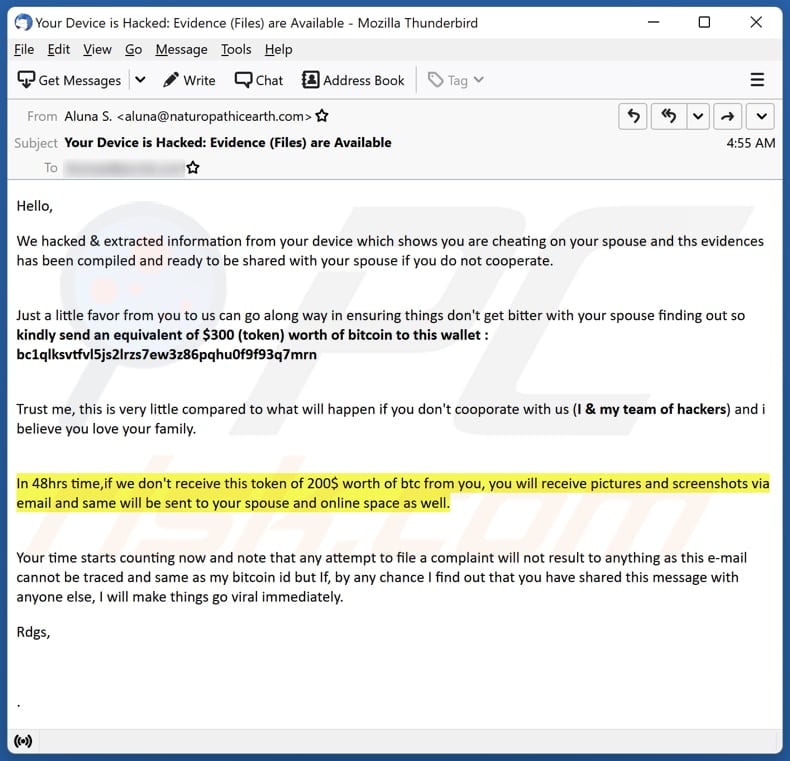In this image, there is a white background framed by a blue outline. At the top, there is a white box with a blue circle icon resembling a person's head, accompanied by the text, "Your device is hacked, evidence files are available, Mozilla Thunderbird." This section also includes a minimize line, a square for maximizing, and a close 'X' button. 

Below this, a blue toolbar displays various menu options: "File," "Edit," "View," "Go," "Message," "Tools," and "Help." Next, a subsequent box features a black box with a down arrow labeled "Get Messages." Adjacent to this are buttons for "Write" (with a pencil icon and a down arrow), "Chat," and "Address Book." Another box includes the "Tag" option with a down arrow and three horizontal lines.

Further down, a blue-highlighted email section shows the sender's details: "From Aluna S, aluna@naturopathicearth.com," marked with one black star. Additional navigation arrows are present in five small boxes, indicating different actions. The email's timestamp reads "4:55 AM." 

The email's subject, "Your device is hacked, evidence files are available," is coupled with a marking indicating it is starred. The body of the email unfolds a phishing scam, claiming the recipient's device has been hacked and evidence of infidelity has been collected. It warns that the information will be shared with their spouse unless they cooperate. 

The hackers demand an equivalent of $300 in Bitcoin to a specified wallet address, emphasizing the urgency by stating that if the payment is not received within 48 hours, incriminating pictures and screenshots will be shared online and with the recipient's spouse. The email is menacingly clear that any attempt to report the issue will be futile and threatens immediate viral exposure if the recipient shares the message with anyone. The email is signed "R-D-G-S," below which a blue line with parentheses and small black marks is visible.